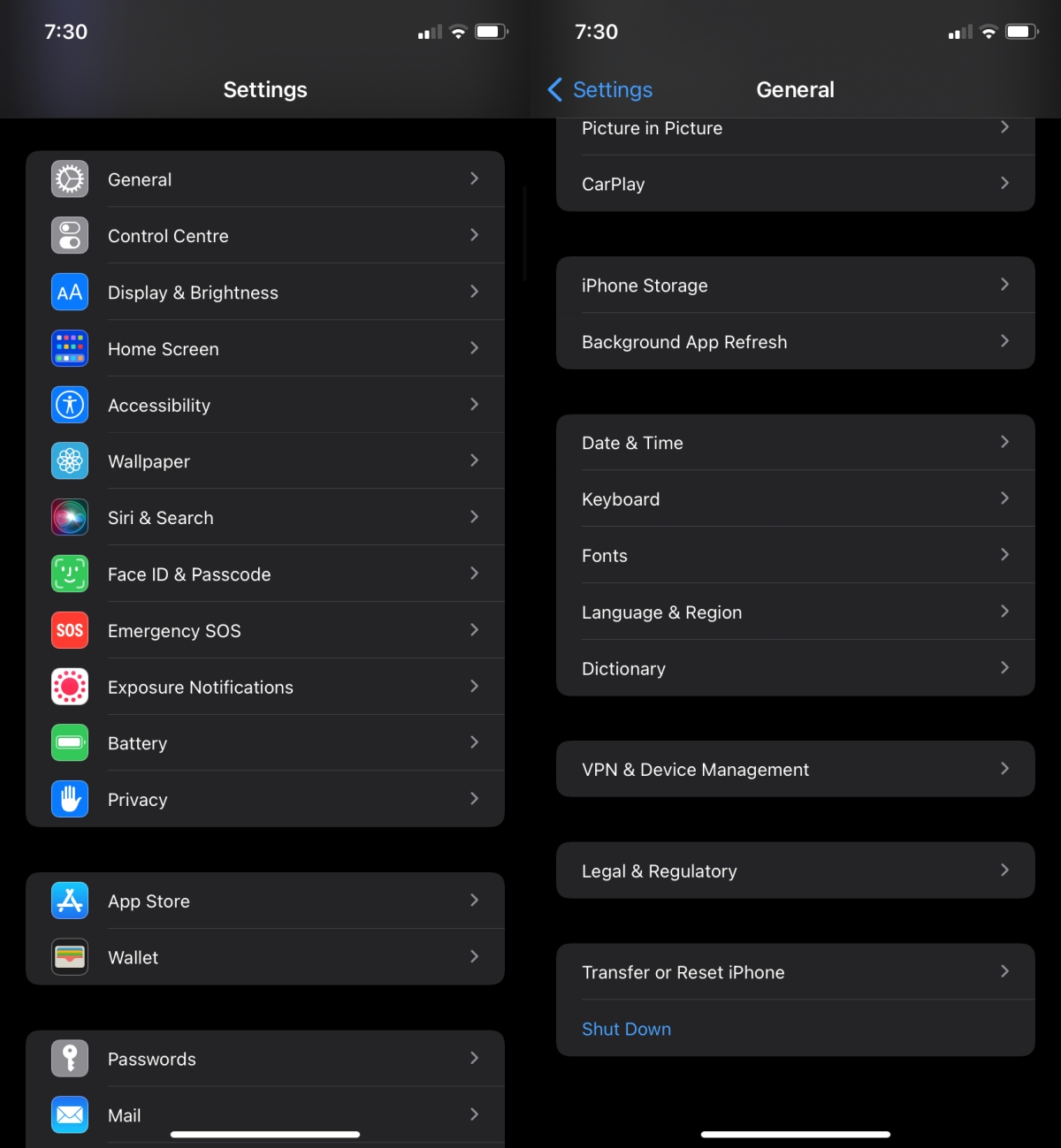A vertical rectangular screenshot of a cell phone's settings menu, predominantly black in the background with grey boxes dividing the content into two columns. The left side of the screen displays the time, "7:30," along with indicators for cell signal (2 bars), Wi-Fi (2 bars), and battery level (three-quarters full). Underneath, various settings options are listed with their respective icons:

- Settings
- General
- Control Center
- Display & Brightness
- Home Screen
- Accessibility
- Wallpaper
- Siri & Search
- Face ID & Passcode
- Emergency SOS
- Exposure Notifications
- Battery
- Privacy
- App Store
- Wallet
- Passwords
- Mail

The right-hand side of the screenshot features another list of settings, indicating specific options available under the "General" section:

- General
- Picture in Picture
- CarPlay
- iPhone Storage
- Background App Refresh
- Date & Time
- Keyboard
- Fonts
- Language & Region
- Dictionary
- VPN & Device Management
- Legal & Regulatory
- Transfer or Reset iPhone
- Shut Down (displayed in blue)

Each section is neatly organized with typical iPhone icons, providing a comprehensive overview of the device's customizable options.